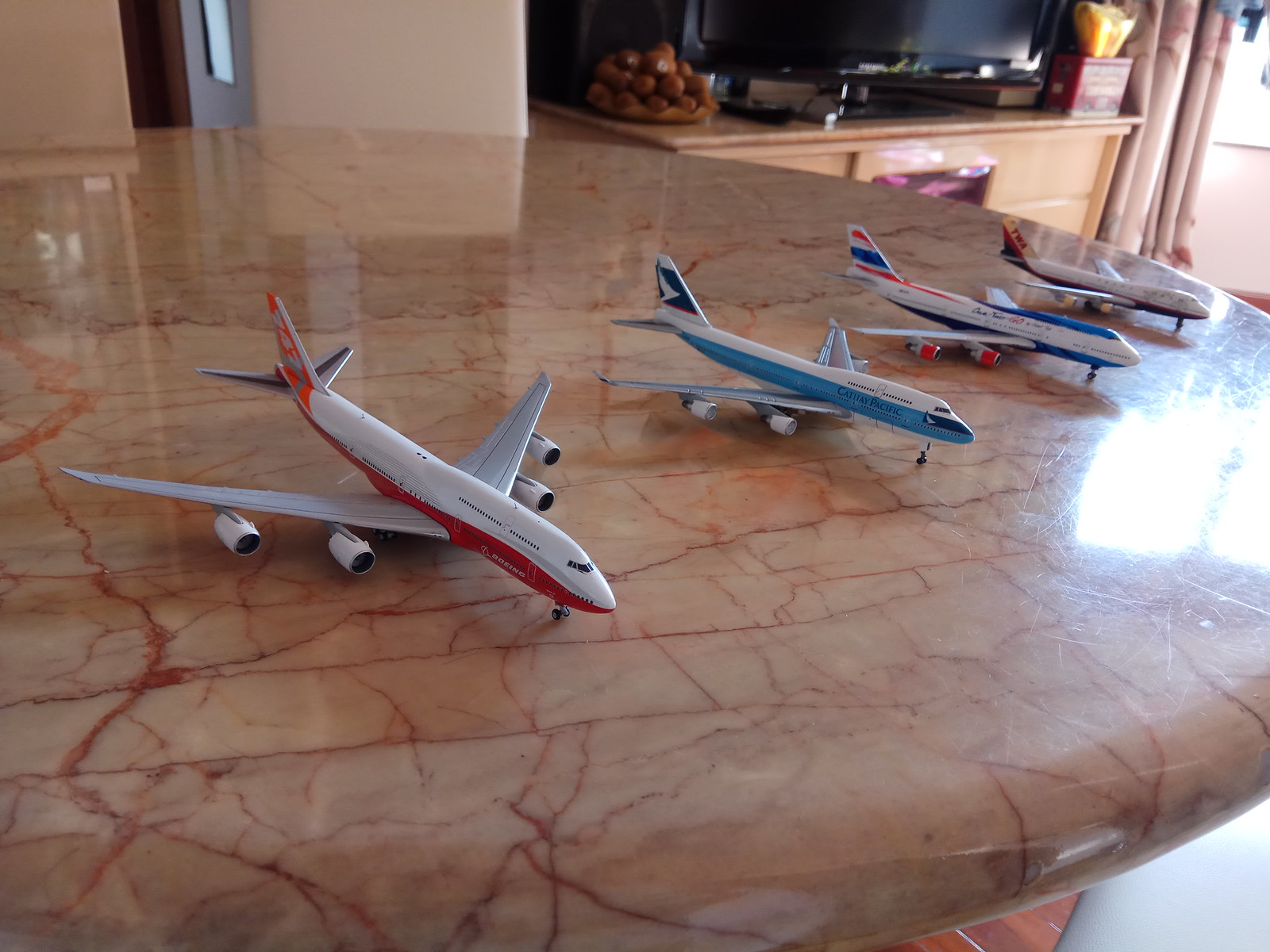This photograph captures a rounded kitchen counter made of tan marble with striking red veins running through it. The countertop showcases a collection of five highly detailed model-sized commercial jet aircraft, specifically 747 types, each bearing distinct livery. The first model is predominantly white, accented with a red stripe along its body. The second model is white with a prominent light blue stripe down the middle. The third displays a blue cockpit area contrasting with its white body. The fourth airplane is entirely white with a brown tail, while the fifth model—visible in some descriptions—appears to have white body markings with nuanced blue and red details. The background features kitchen elements including a wooden cabinet topped with a television, adding context to the realistic kitchen setting.